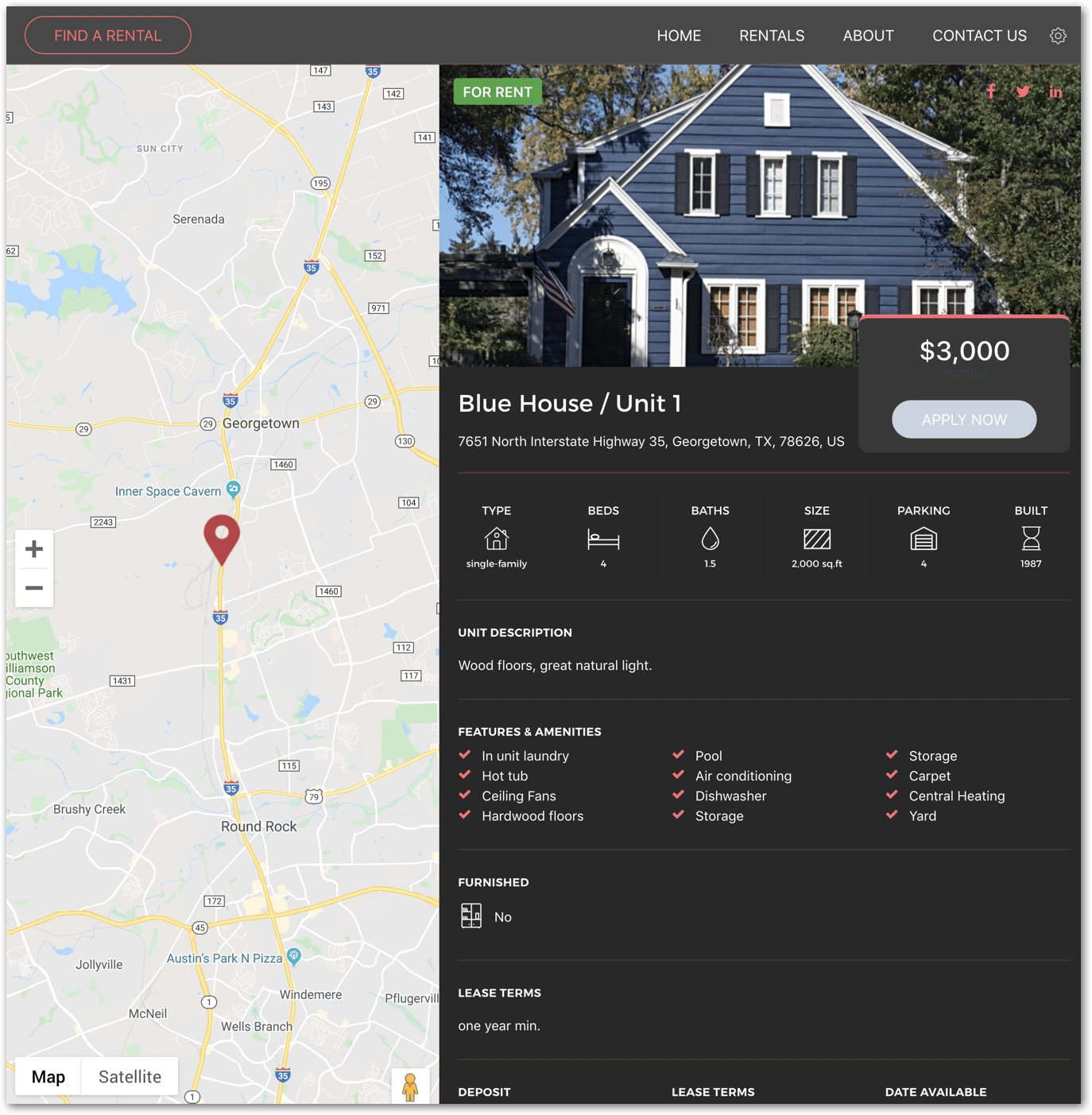This cropped screenshot showcases the desktop version of a home rental website. The site features a predominantly black header with a red-outlined circle, prominently displaying the phrase "Find a Rental" in bold red font. On the right side of the header, options such as "Home Rentals," "About," and "Contact Us" are presented in bold white font, accompanied by a cogwheel icon for settings on the far right.

The main content of the page is divided into two sections. The entire left side is occupied by a map with a central pin drop indicating the location. The right side features a detailed listing for a house. At the top of this section, a photo of a blue house with a prominent green "For Rent" sign is displayed. In the bottom right corner of the listing section, a black box with a red horizontal line at the top reveals the rental price: $3,000, presented in large white numbers, and a blue "Apply Now" button just below it.

Underneath the house photo, the listing provides the basic information: "Blue House Unit 1," followed by the address in small white letters. Below this, a horizontal line of icons offers further details about the property. Categories such as "Type," represented with a house icon and labeled "Single Family," are shown, followed by "Beds," depicted with a bed icon but not listing the number of beds. Additional categories like "Bath," "Size," "Parking," and "Built" also appear, but their specific details are not provided.

The "Unit Description" section follows, offering a brief summary of the property. Beneath this, the "Features and Amenities" section lists various features, each highlighted by red check marks. Further down, the screenshot indicates "Furnishings," which is marked as "No," and "Lease Terms." The screenshot cuts off at the bottom, leaving some details hidden.